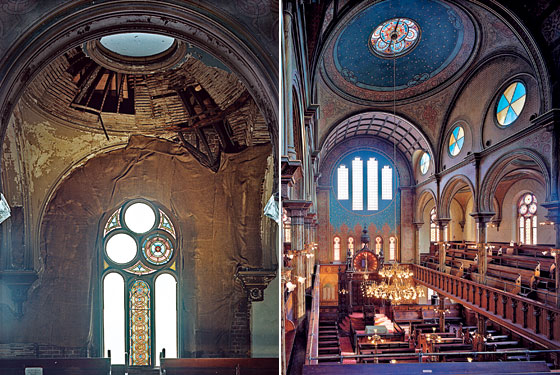Two side-by-side photographs showcase the interior of churches with high, arched ceilings and intricate stained glass windows. The left image depicts a decayed church with an arched dome ceiling in disrepair, areas where wood rafters have been stripped away, and clear skylights exposed to the open air. The stained glass in the lower arched window is partially intact, while other sections have clear glass. Paint is peeling, and the roof appears to be partially missing, exposing the rafters overhead. Empty pews line the floor, creating a sense of abandonment. 

In contrast, the right image presents a restored, pristine church interior viewed from a loft. The arched domes and stained glass windows are immaculate, with vibrant colors and detailed designs. Rows of pews are perfectly aligned, and a few people may be seen seated. A set of steps leads up to a prominent podium, hinting at the active use of the space. This could be a before-and-after comparison highlighting the transformation from dilapidation to restored grandeur.